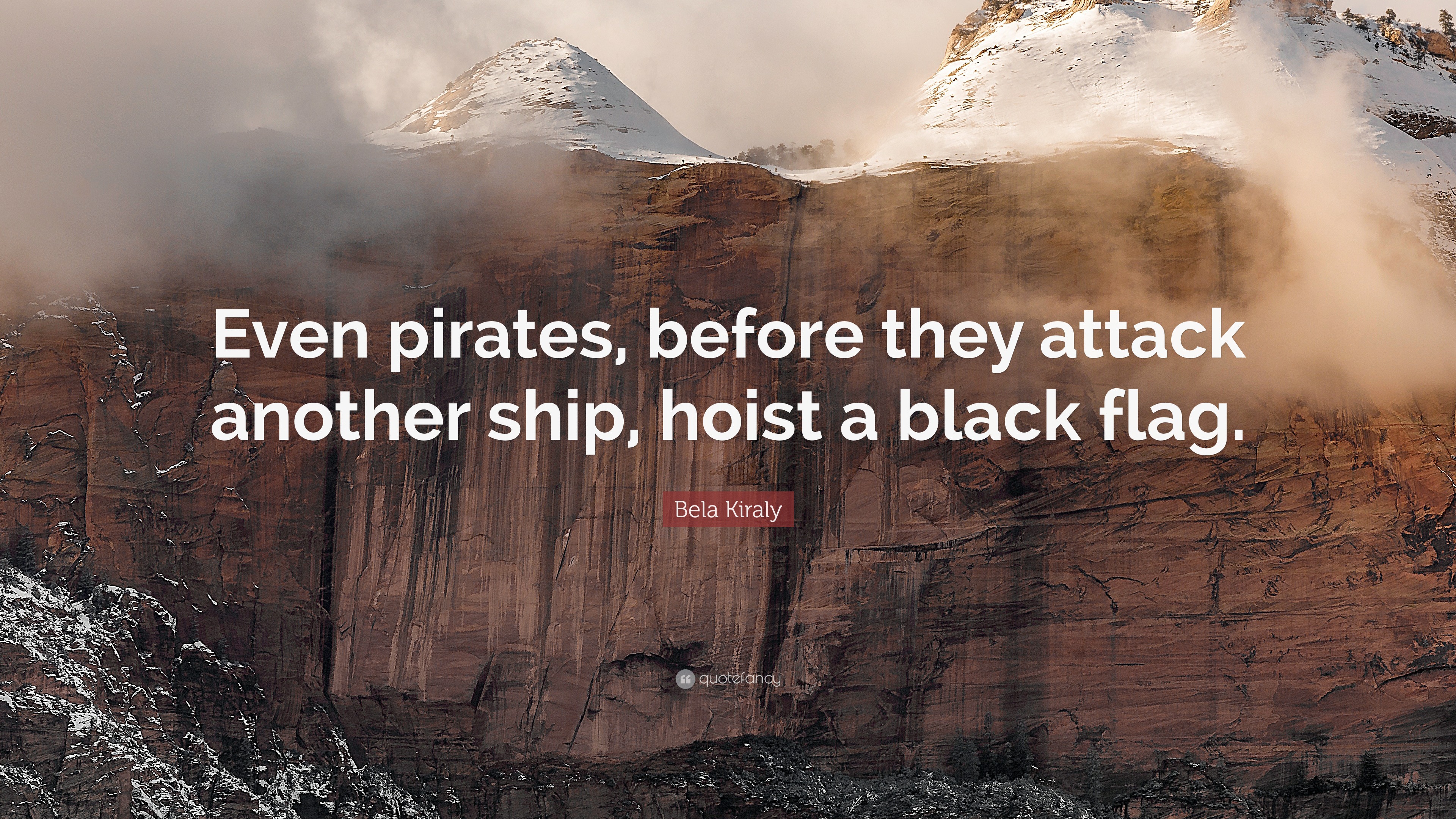The photograph showcases a high-altitude mountainous landscape featuring a striking brown cliff face that appears as though it has been cut flat vertically. Dominating the frame, the cliff stretches almost from the top to the bottom of the image, with snowy, triangular mountain peaks visible behind it. The sky is filled with a mix of clouds and fog, suggesting a foggy day, and the mist partially obscures the cliff face along the left and right edges. In the center of the image, there is a white text overlay that reads, "Even pirates, before they attack another ship, hoist a black flag." Below this quote, a smaller red rectangular box contains the white text, "Bella Kiraly." The photograph appears to capture not only the rugged beauty of the mountainous terrain but also serves as a possible advertisement, given the prominent placement of the quote and name.